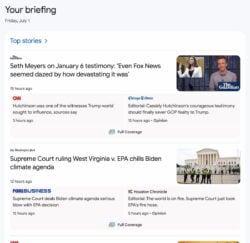This image is a cropped screenshot of a "Your Briefing" page from a news app. The background is an unembellished gray, adding a minimalist touch to the interface. The top of the screenshot prominently features the heading "Your Briefing" in bold lettering. Directly beneath this heading on the left side, the date is displayed in small, unobtrusive text. 

Dominating the center of the image is a large white overlay box, contrasting starkly with the gray backdrop. Inside this box, in the top-left corner, the label "Top Stories" is displayed along with a leftward pointing arrow, indicating navigation options. 

Listed below this are various news stories, aligned horizontally. The first headline is sourced from The Guardian website, followed by articles from CNN, NBC News, and a final section labeled "from Business" which sits just above a centered button. This button is labeled "Full Coverage," inviting users to click for more detailed stories.

Additionally, two thumbnail images are positioned on the right side of the story titles, providing a visual cue to accompany the text headlines.